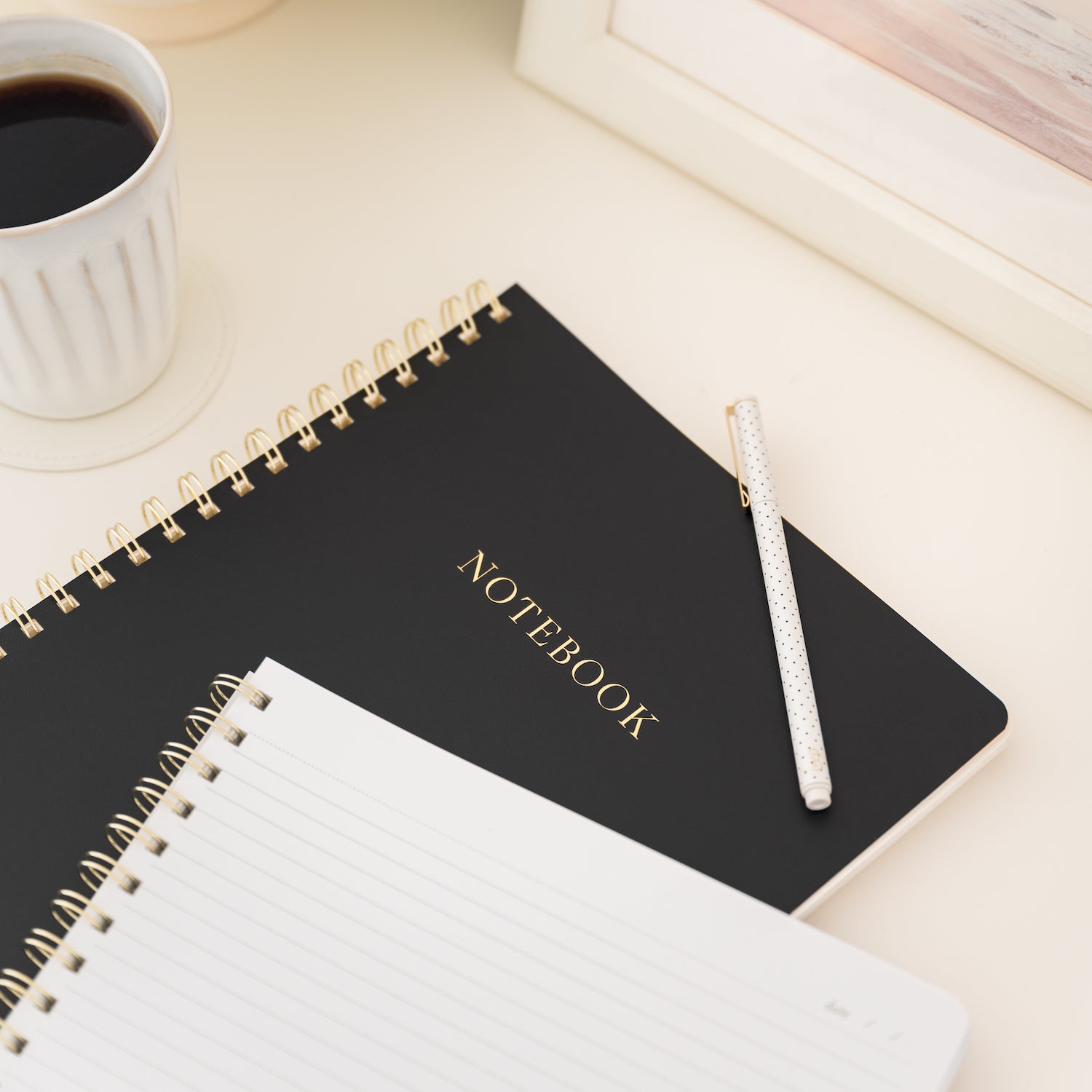This detailed color photograph captures an intimate desk area scene. In the upper left-hand corner, a white coffee cup, partially filled with coffee, rests on a matching white saucer. This setup is placed on a pristine white surface, which could be a desk or countertop. Nearby, the bottom left corner of a framed print is visible, featuring shades of pink, gray, pale purple, and white. In front of this frame, there is a black notebook with a gold spiral binding, prominently displaying the word "NOTEBOOK" in gold, all-caps lettering. A white pen with speckles and a gold clasp lies diagonally across the top of this closed notebook. Adjacent to it, an open spiral-bound notebook reveals lined white pages, with its cover folded back. Both notebooks and the pen rest on the same smooth, white surface, creating a unified and minimalistic workspace aesthetic.